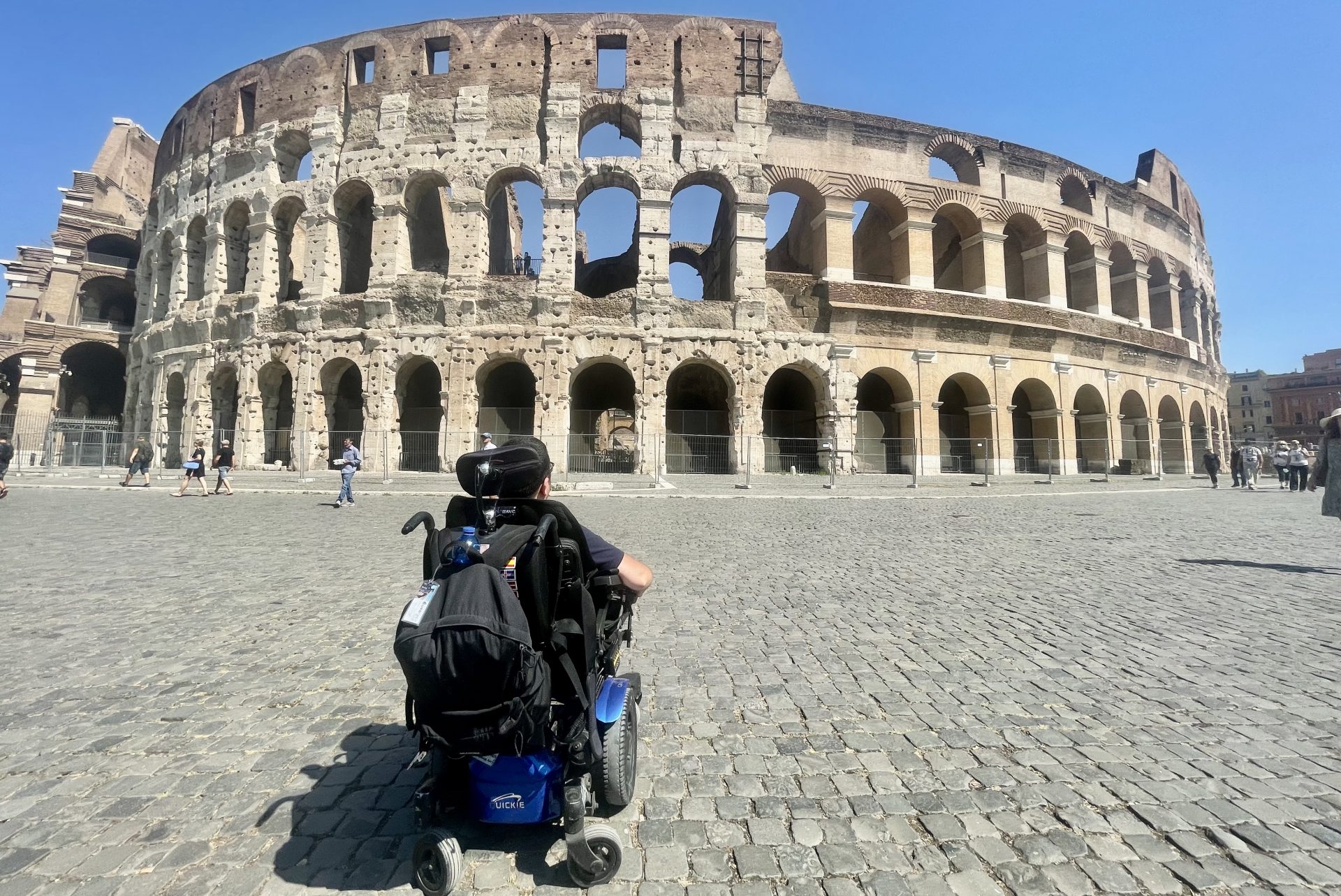The image is a color photograph of the iconic Colosseum in Rome, captured from the outside on a bright, cloudless day with a vivid blue sky. The ancient stone structure boasts three levels of archways, with the left side displaying a rougher, pockmarked texture characteristic of its ancient origins, while the right side appears smoother and more reconstructed. The ground in front of the Colosseum consists of gray cobblestone paving, with a wide open area extending towards the viewer. In the foreground, there is a black and blue electric wheelchair with a large black backpack hanging from its back, occupied by a person viewed from behind, revealing an elbow, the back of an ear, and dark hair peeking out from a black t-shirt. The scene includes a few distant pedestrians walking near the fenced base of the historic amphitheater.